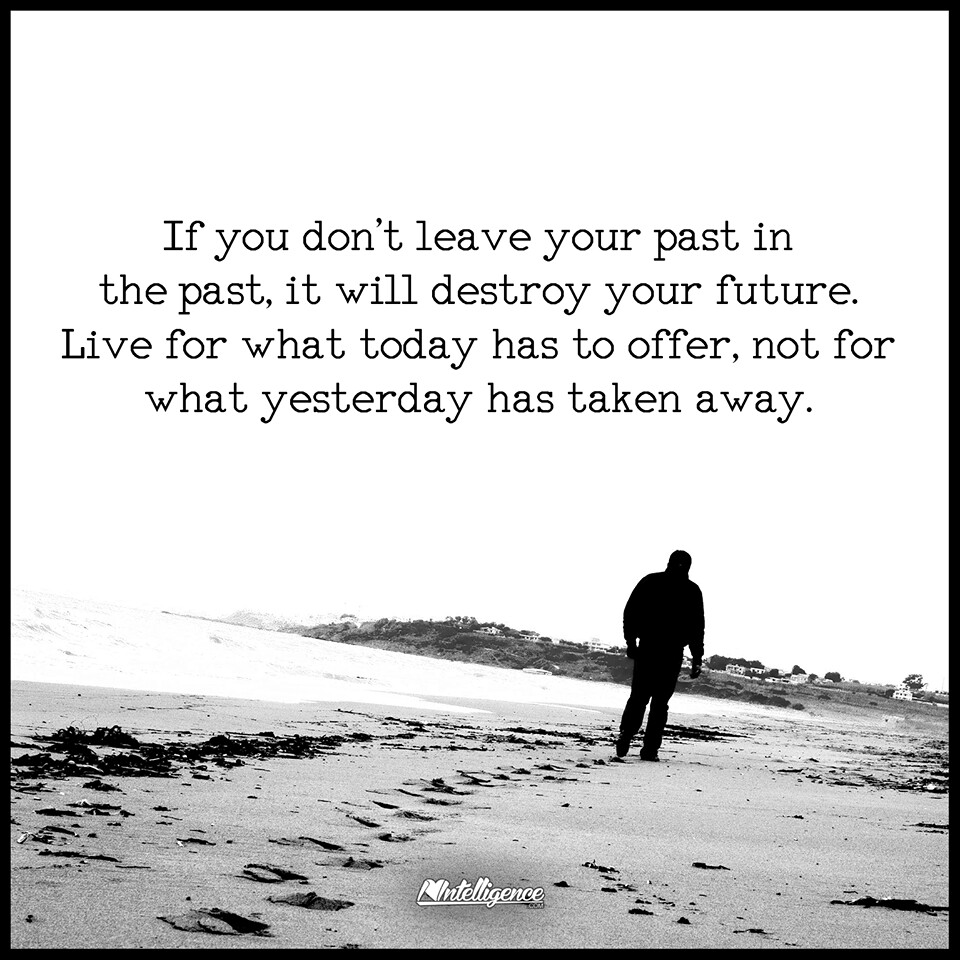The black and white image portrays a man walking alone along a beach, moving away from the camera's perspective. His footprints trail behind him in the sand, with gentle ocean waves lapping at the shore to his left. In the distance, a small peninsula extends out to the left, dotted with houses and some trees. A blocky, courier-like font displays an inspirational quote in black text over the image, reading: "If you don't leave your past in the past, it will destroy your future. Live for what today has to offer, not for what yesterday has taken away." Encircling the photograph is a thin black line framing it, and at the bottom center, the word 'Intelligence' is written with a white underline.